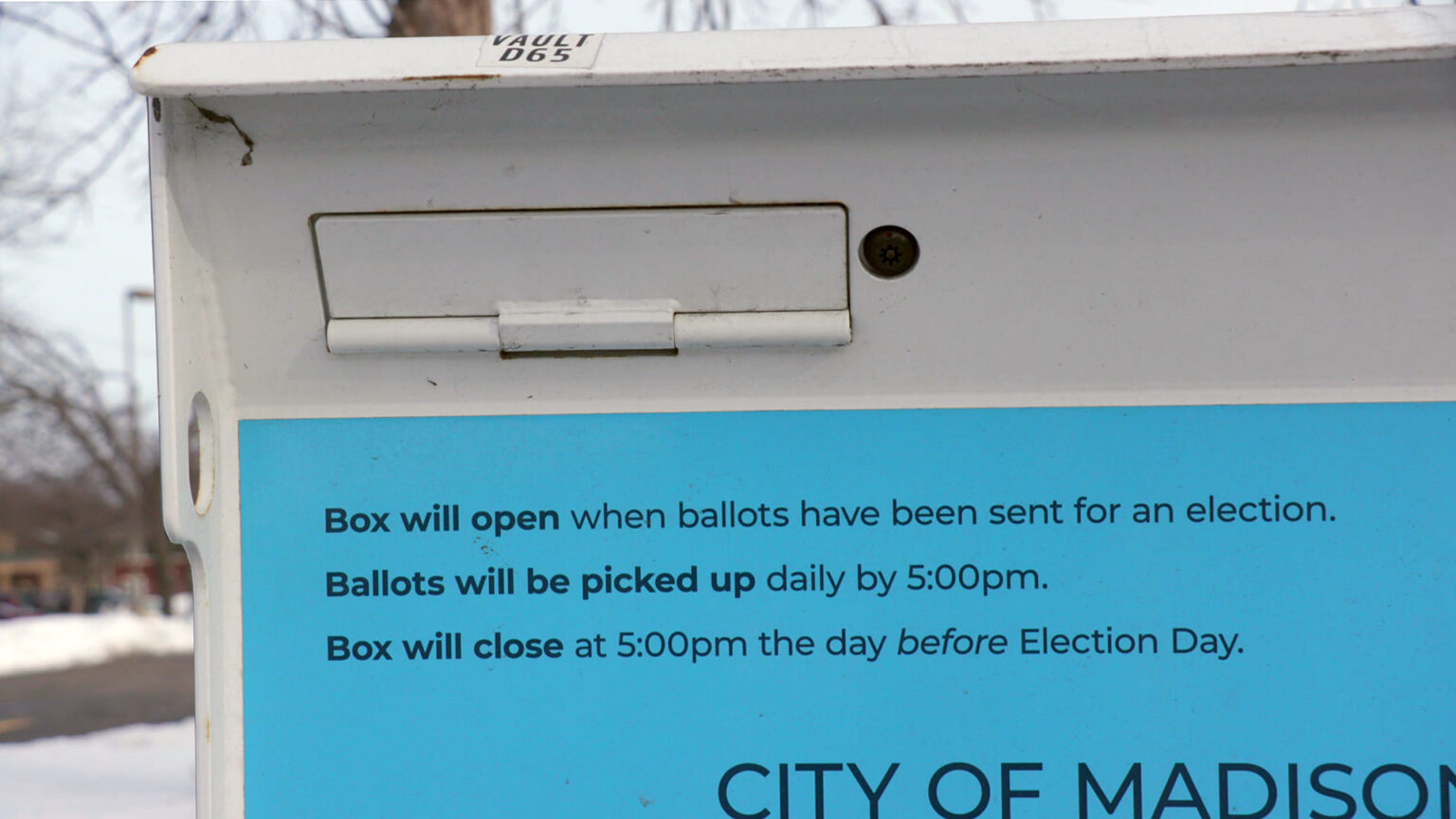This photograph is a close-up image of the upper left portion of a white ballot box, with only the top and left edges revealing a blurry, snowy background that includes bare trees and possibly a telephone or light pole. The top of the ballot box features a sticker reading "Vault D65," with a keyhole adjacent to a slot designed for ballot insertion. The ballot box itself extends off the right edge of the photo, obscuring its full shape and size. Prominently displayed on the front of the box is a large blue sign with detailed instructions in black text, stating: "Box will open when ballots have been sent for an election. Ballots will be picked up daily by 5 p.m. Box will close at 5 p.m. the day before Election Day." In the bottom right corner of the box, partially cut off by the edge of the image, are the words "City of Madison," with the last letter "N" not fully visible.